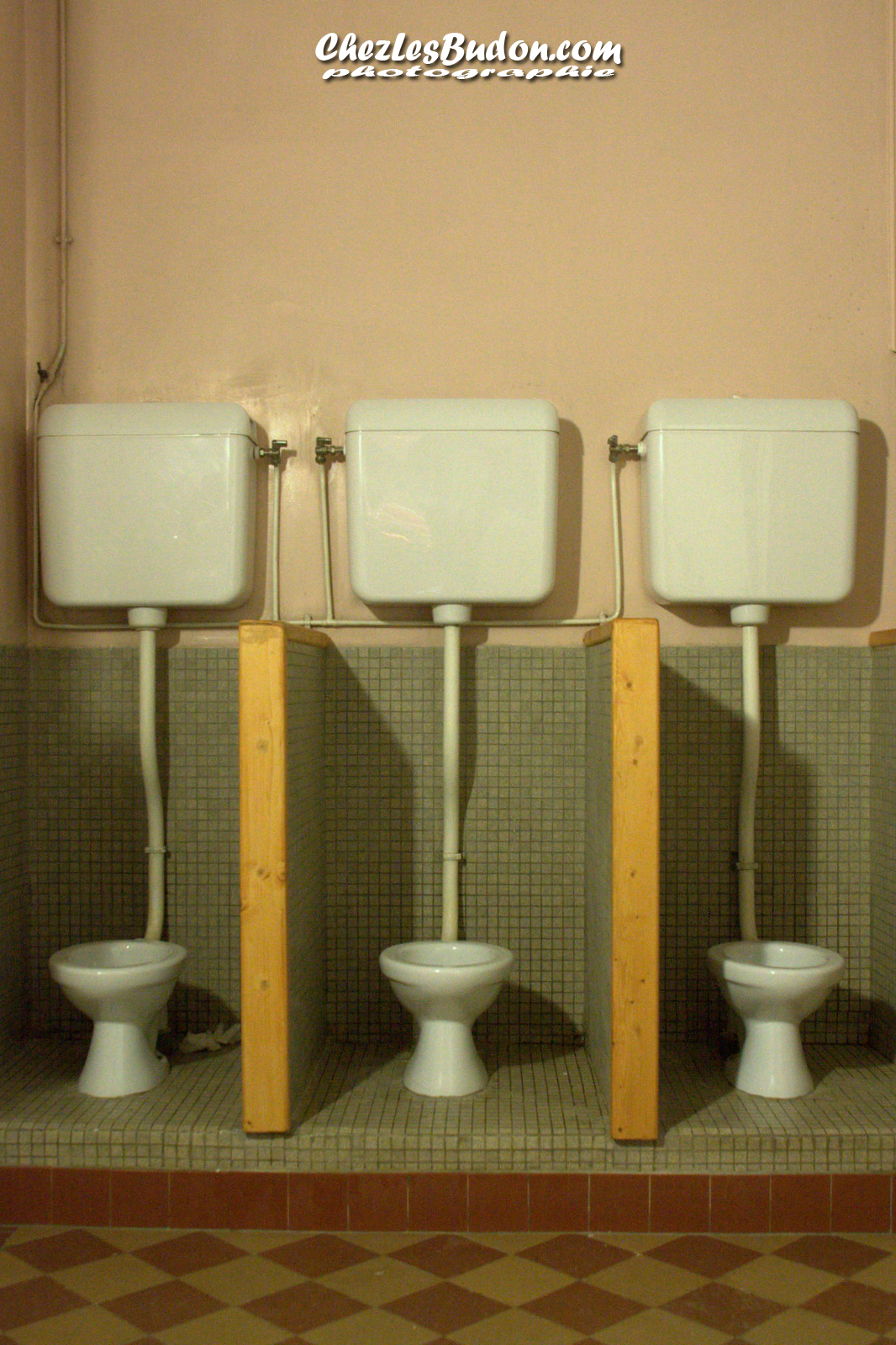This image showcases a vintage-inspired bathroom with three distinct open stalls, each separated by low wooden-framed partitions. The stalls feature old-fashioned high-tank toilets with white porcelain bases and long connecting pipes. The toilets, notably lacking seats and lids, are set against a backdrop of small dark green tiles that ascend halfway up the wall of each stall. Above, the wall is cream-colored, featuring the text "charlesboudon.com" followed by "photography" in white font at the top of the image. The stalls are arranged on an elevated step bordered by red tiles, contrasting with the brownish-gray small tiles within each stall. The main floor is decorated with an eye-catching red and gold checkerboard pattern, contributing to the restroom's distinctive aesthetic.